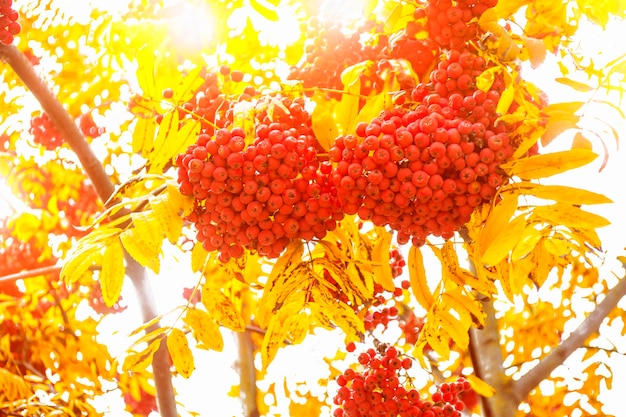The vibrant image showcases a close-up view of a tree adorned with clusters of bright red, pea-sized fruits that resemble miniature tomatoes or berries. These fruits, grouped together like bunches of grapes, emerge prominently from the tree, with each fruit having a small stem or stub at the top, akin to a tomato. Yellow leaves surround these red clusters, contributing to the tree's colorful display. The tree, possibly a raspberry bush given the appearance of the fruits, features a light green bark that begins from the lower right corner, extending upwards into the yellow foliage. Additional stems, rising from the lower left and towards the center, also support the yellow leaves and vibrant red fruits. The background highlights a bright sky with sunlight illuminating the scene, enhancing the vividness of the colors and the overall clarity of the image. This detailed and well-lit outdoor setting captures a strikingly beautiful and eye-catching moment.